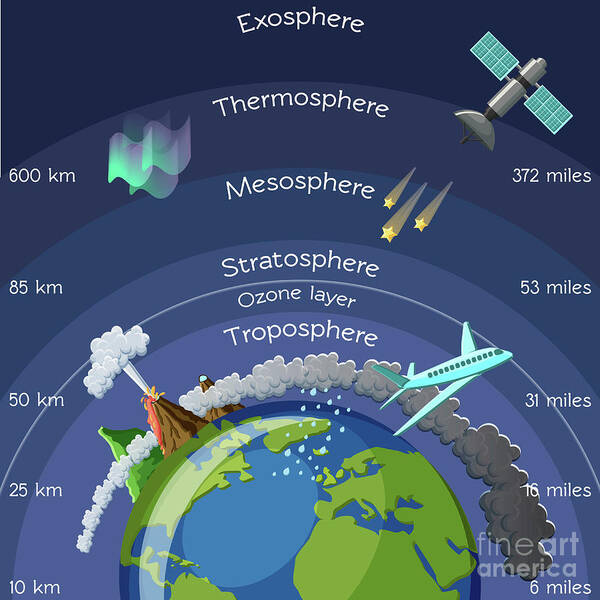This detailed drawing illustrates the different layers of Earth's atmosphere, styled in a way that is both scientific and accessible, reminiscent of children's educational material. The scene is set in space, showcasing a semicircle of the planet Earth with visible landmasses—North and South America, parts of Europe, and half of Africa—colored in green, while the water bodies are depicted in blue. Clouds adorn the troposphere, and a volcano is located near North America. An airplane is illustrated flying away from Europe within this layer.

Elevation markers on the left side of the image list heights in kilometers: 10 km, 25 km, 50 km, 85 km, and 600 km, while on the right side, the corresponding heights are given in miles: 6 miles, 16 miles, 31 miles, 53 miles, and 372 miles. The atmospheric layers are labeled from the bottom up: troposphere, stratosphere, ozone layer, mesosphere, thermosphere, and exosphere. The troposphere, home to most weather phenomena, extends up to 6 miles or 10 kilometers, and features both the volcano's clouds reaching into the ozone layer and the airplane in flight.

Above the troposphere lies the ozone layer within the stratosphere, which goes up to 31 miles or 50 kilometers. The mesosphere extends further up to 53 miles or 85 kilometers and is marked by shooting stars where meteorites burn up. Above all these is the thermosphere, home to phenomena like the aurora borealis and extending up to 372 miles or 600 kilometers, with a satellite depicted in the exosphere in the top right corner.

Additional elements include three stars situated to the right of the stratosphere label, northern lights in the top left corner, and a watermark labeled "Flying on America" in the bottom right corner. The meticulous details and clear segmentation of atmospheric layers make this a comprehensive diagram of Earth's atmospheric structure.